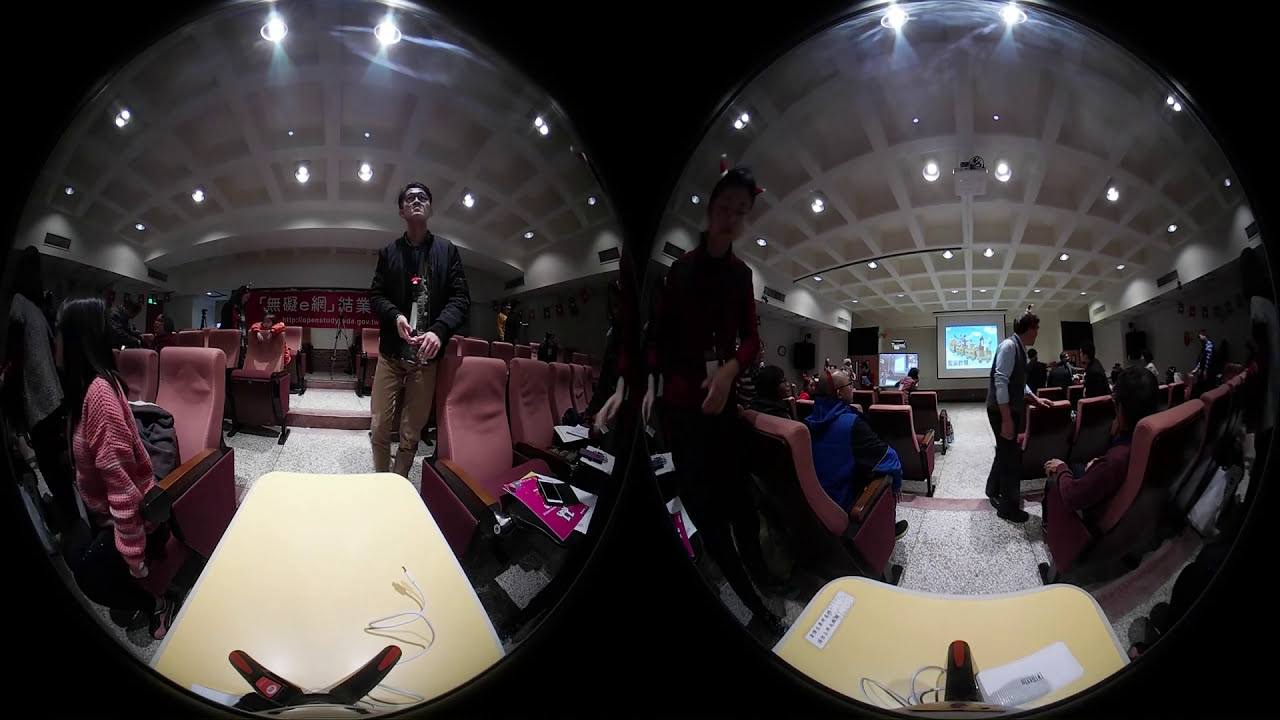The image shows a slightly distorted, double-circular view of a mini movie theater with red, comfortable cloth seats. Each circle presents a different angle of the same room. The right circle features a beige or yellow rectangle mouse pad with a white sticker and possible black letters, along with a thin white cord. The red chairs, arranged in rows, face a projector screen at the far end of the room, surrounded by scalloped white walls and ceiling lights. In the left circle, a man in a black jacket stands in the center aisle, heavily shadowed, next to a woman with long black hair wearing a red striped shirt. The fold-out tables in front of the seats are clearly visible, and people appear to be discussing something, possibly related to a previous or upcoming screening. The movie screen at the back shows a combination of red, blue, and white colors.